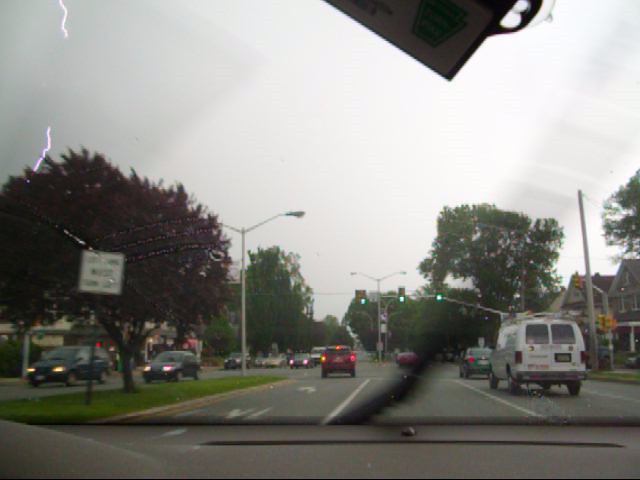The photograph captures a dynamic street scene on a cloudy day. In the left-hand corner, two vivid lightning bolts streak across the sky, one at the top of the frame and the other near the edge of a tree adorned with reddish leaves. The street is bustling with traffic, and all the visible traffic signals display green lights. Among the vehicles, a gray car with its headlights on is heading towards the viewer. A white service minivan, marked with writing but without its lights on, is also present. In addition, a red pickup truck drives ahead, its taillights glowing. The image is shot from the inside of a moving car, evidenced by the windshield wiper caught mid-swipe in the frame.